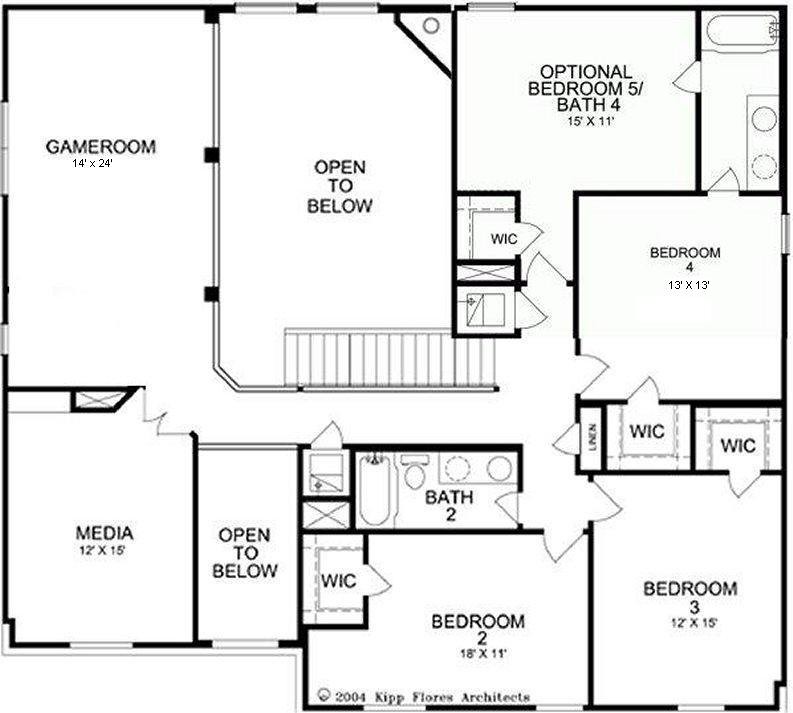This is a detailed floor plan diagram of an expansive, single-story home, showcasing a thoughtful layout with a variety of rooms catering to different needs. Starting in the top left corner, the first room is a spacious game room, perfect for recreational activities. Directly below the game room is a media room, ideal for entertainment and movie nights. To the right of the media room, there's an open area leading to the lower part of the home. 

In the top right corner, there are four bedrooms strategically positioned for comfort and privacy. Two bedrooms are located side-by-side in the right top corner, with another bedroom situated in the middle of the right wall. The top right corner features an optional fourth bedroom, providing flexibility for use as a guest room or home office.

This upper floor plan also includes several bathrooms to accommodate the needs of its residents. A stairway is present, leading down to additional living spaces, indicating a multi-level home. This extensive and well-designed home offers multiple rooms such as bathrooms, washrooms, and essential living areas, ensuring all functional requirements for comfortable living are met.